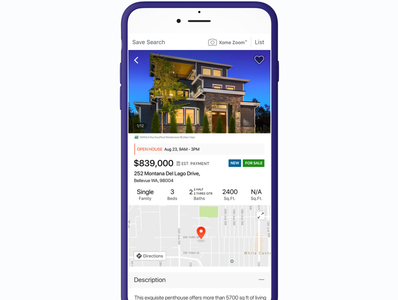The image features a light blue background with a purple smartphone interface prominently displayed. At the top of the screen, there is a "Save Search" option, followed by icons that include a small square and a list. A left arrow is also visible. The main section of the screen showcases a vibrant photo of a beautiful three-story house against a blue background. In the upper right corner of the photo, there is a small black heart icon. Below the picture, a white block displays the price of the house, listed at $839,000. Next to the price, there is a blue "New" button and a green button. The property is described as a single-family home containing three bedrooms, two bathrooms, and covering 2,400 square feet. Additionally, a small blue map with a red pin indicates the location of the property. Below the map, there is a description box, followed by another line of text that gets cut off.